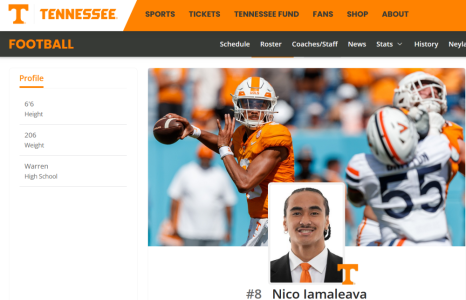The image is a detailed portrayal of Tennessee football's website or promotional material. At the top, a large orange "T" prominently marks the Tennessee logo, followed by the word "Tennessee" beneath it, all set within a rectangular white background. Black print headers mark categories such as "Sports," "Tickets," and "Tennessee Fund," with additional sections labeled "Fans," "Shop," and "About."

The next section features the word "Football" in bold orange letters against a black background, with white text categories like "Schedule," "Roster," "Coaches/Staff," "News," "Stats," and "History." The word "Nay" is partially visible but cut off, indicating incomplete text.

A profile section below details a player, listing height as 6'6", weight as 206 lbs, and "Warren High School." The focus is on a player wearing number eight, identified as Nico Amamalava. He is shown smiling in a photograph, dressed in a suit coat, dress shirt, and an orange tie, with a "T" beside his image. In the background, another image depicts him throwing a football.